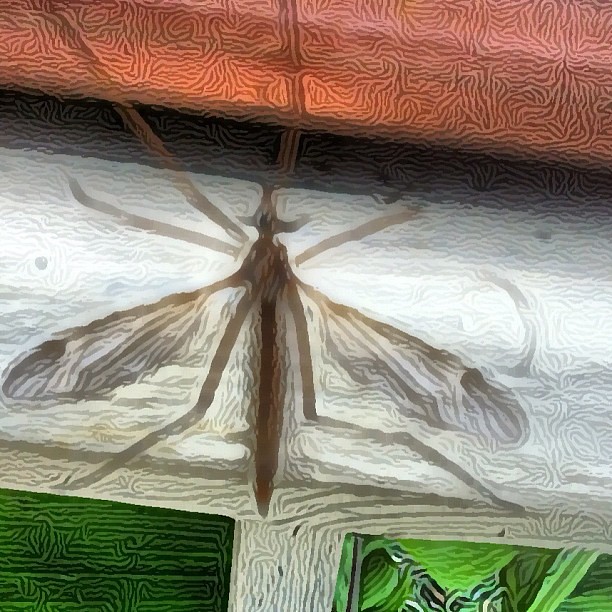This artwork appears to be a unique and intricate drawing with a captivating blend of colors and lines. Dominating the center of the image is a detailed depiction of a large mosquito in brown, characterized by its wings, elongated body, and prominent legs. The background composition showcases a series of vibrant and contrasting colors: the top features a gradient from reddish-pink to dark red squiggly lines, adding a sense of dynamic movement. Below these lines, there's a distinct horizontal black line, transitioning into areas of white, gray, and tan that create a layered effect. Toward the bottom, two green squares are present, anchoring the composition and enhancing its overall balance. The mosquito appears artfully rendered, blending seamlessly into this complex backdrop, making it challenging at first to distinguish whether it is real or an impressively drawn figure.